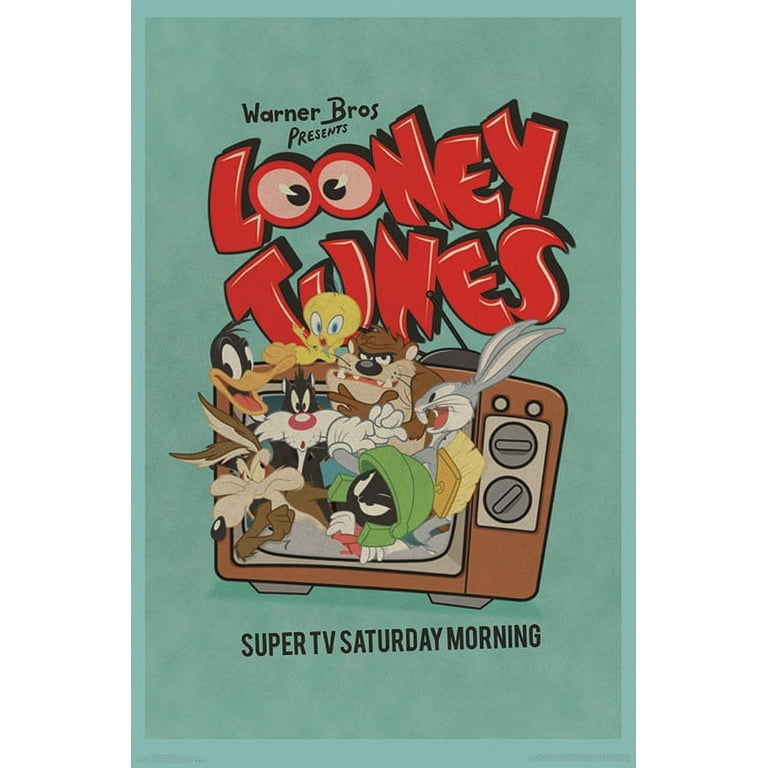The image depicts a nostalgic advertisement for Looney Tunes on a faded turquoise vertical rectangle on a white background. At the top, in small black letters, it says "Warner Brothers presents." Below this, in large, playful red letters, "Looney Tunes" is prominently displayed, with the two O's cleverly designed as crossed pink eyeballs with black pupils. Underneath this title, a brown, vintage television with knobs, little legs, and an old-fashioned antenna takes center stage. Emanating from its screen are beloved Looney Tunes characters: Wile E. Coyote, Daffy Duck, the Tasmanian Devil, Tweety Bird with a surprised look, Bugs Bunny sporting a mischievous grin, Marvin the Martian, and Sylvester the Cat. At the bottom, in small dark letters, the text reads "Super TV Saturday morning,” completing this vibrant and inviting scene.